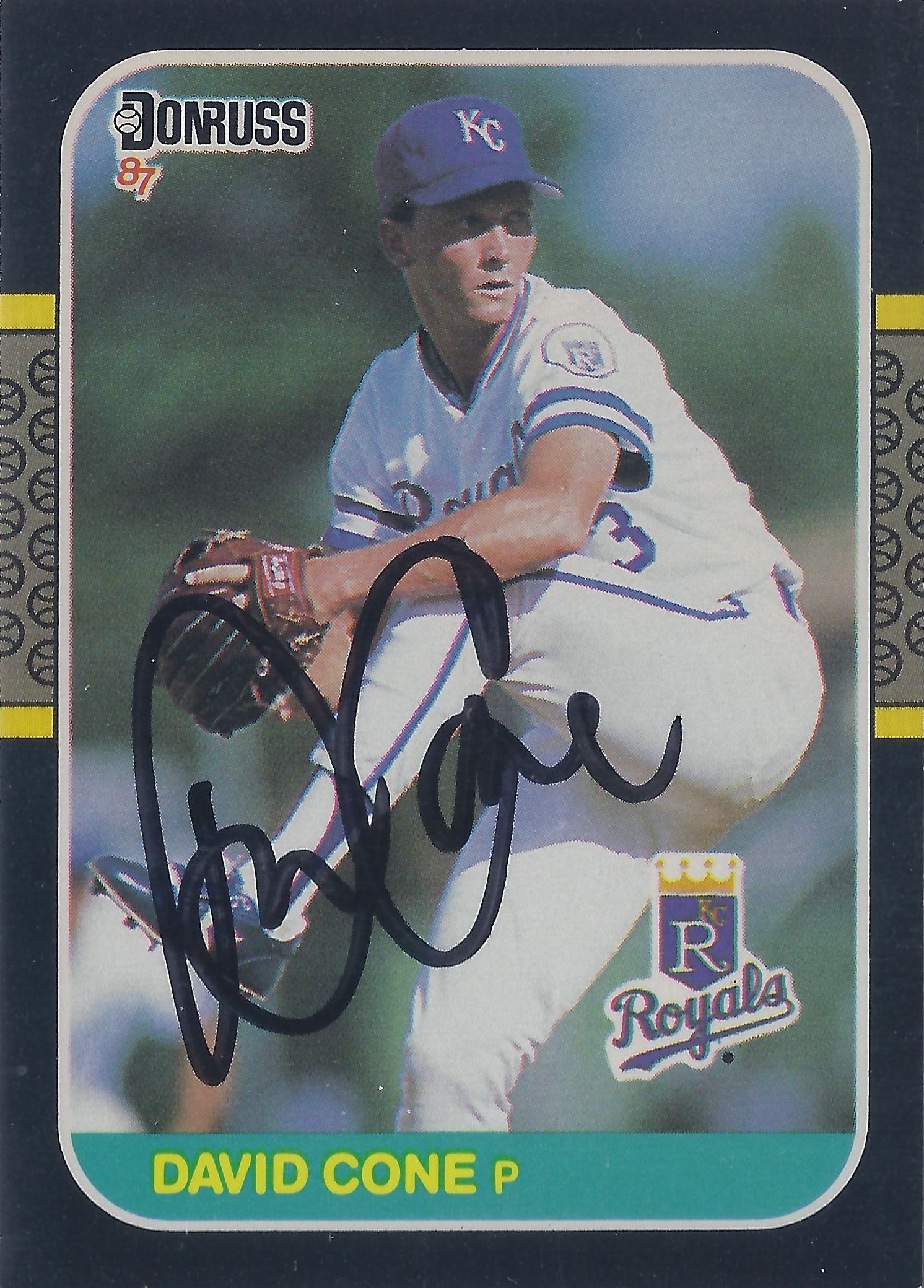The image is a close-up of a vintage 1987 Donruss baseball card, featuring pitcher David Cohn from the Kansas City Royals. The card is rectangular with a black border and has silver and yellow strips with black-outlined baseballs at the ends. At the top left, the card is labeled "Donruss '87." A yellow crown is also present at the top. 

The centerpiece of the card showcases a dynamic image of David Cohn in mid-pitch. He is dressed in the iconic Kansas City Royals uniform, which consists of a white short-sleeved jersey adorned with blue stripes on the sleeves and the word "Royals" written in blue across the front. His uniform number, partially visible, appears to be three. Cohn is wearing white pants with a blue stripe down the side, white socks with matching blue stripes, and black cleats. His blue cap features the white initials "KC," and he is gripping a brown mitt with one of his hands.

Near the lower left-hand corner of the card, the player's name, "David Cohn," is printed in yellow letters inside a small green box, accompanied by a yellow "P." Adjacent to this, there is a signature made with a black Sharpie, signifying an autograph. The bottom right corner bears the blue "Royals" logo, reinforcing the team identity. The overall design elements and attire suggest the card's vintage nature, from around 1987.